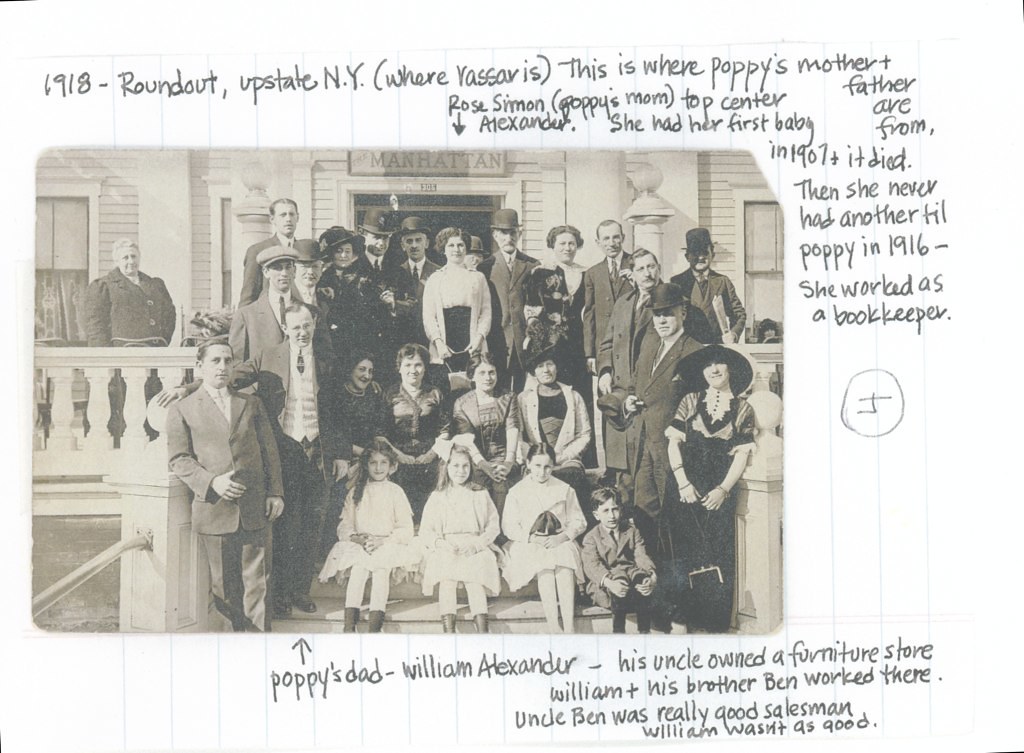This black and white photograph, taken in 1918 in Roundout, Upstate New York, captures a large family gathering in front of a white house with a sign that reads "Manhattan." The family is dressed in early 1900s attire; the men predominantly wear suits, some with neckties and black top hats, while the women are in dresses, with some also wearing hats. 

Written in pencil at the top of the photograph is "1918, Roundout, Upstate New York, where Yasser is. This is where Poppy's mother and father are from." An arrow points toward the top center of the image, identifying Rose Simon Alexander, Poppy's mother. Rose, a bookkeeper, had her first baby in 1907, but sadly, the child did not survive. She did not have another child until Poppy in 1916. 

Toward the bottom, another arrow points upwards to Poppy's father, William Alexander. Noted beside him is a brief family history: William and his brother Ben worked at their Uncle Ben's furniture store, where Ben excelled as a salesman while William struggled.

Right up front in the image, four children—three girls and a boy—are clearly visible among many adults, providing a glimpse into the multi-generational family during that era.